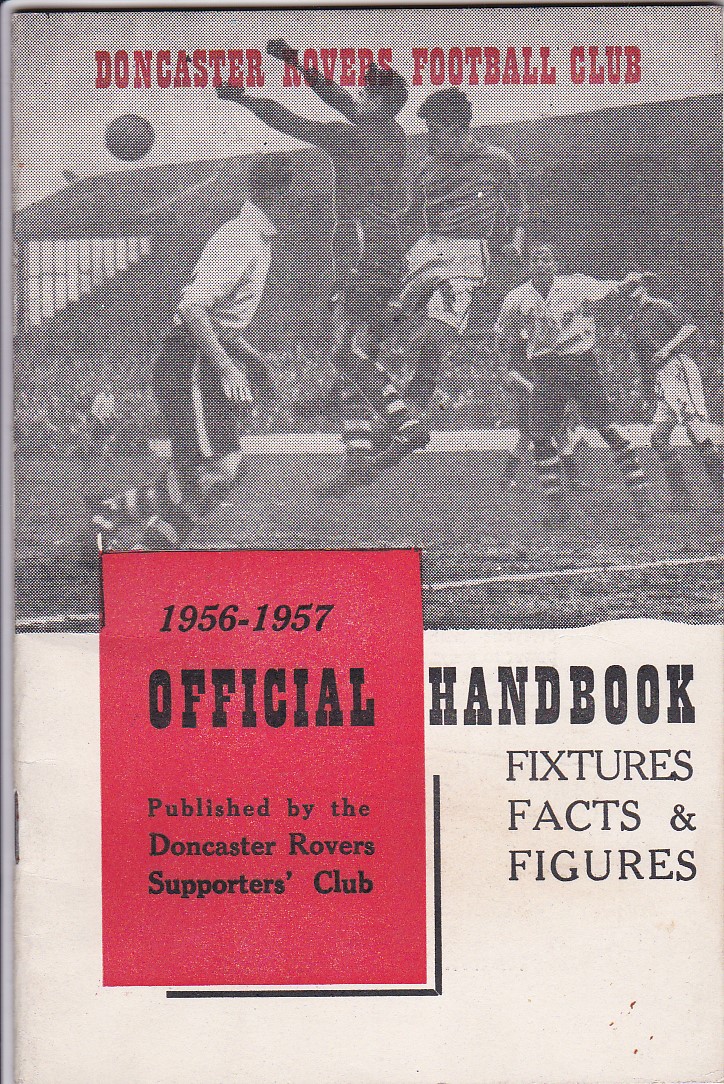This image depicts the 1956-57 Official Handbook of the Doncaster Rovers Football Club, published by the Doncaster Rovers Supporters Club. The cover is divided into two primary sections. The upper half features a grainy black and white photograph of a soccer match, capturing the dynamic action of five players contesting for the ball, with some figures airborne and the stadium stands filled with spectators in the background. The photo shows players in black and white striped socks, enhancing the retro feel of the image. Above this scene, the title "Doncaster Rovers Football Club" is prominently displayed in red lettering. 

The lower half of the cover is more text-centric, with a red rectangle containing the dates "1956-57" and the word "Official" in black text, creating a stark contrast. Below this, the words "Handbook, Fixtures, Facts, and Figures" are printed in black on an off-white background, providing a clear and structured layout of the book's contents. The overall design merges nostalgic imagery with practical information, reflecting the handbook’s purpose and the era in which it was published.